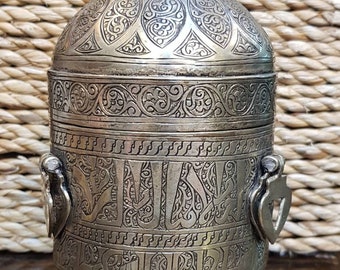An antique container is showcased in a highly zoomed-in photograph, emphasizing the intricate details. The bottom edges feature a lock or tag resembling a shield with a cutout center. The container's surface is adorned with various engraved patterns, including lines, swirling motifs, and intermittent horizontal bands, creating a richly textured appearance. The background is a light tan, quilt-like fabric, accentuating the container's details. The bottom left and right corners of the image are dark brown, providing contrast to the overall light background.